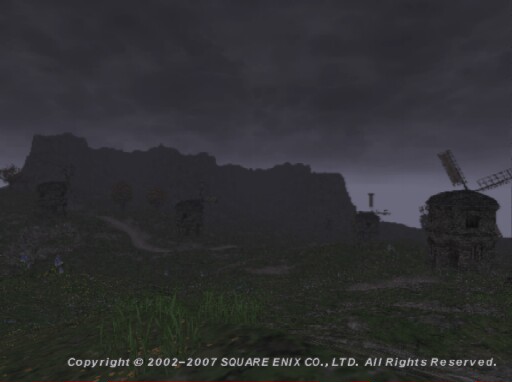This image appears to be a screenshot from a video game, with copyright attributed to Square Enix Co., Ltd., spanning the years 2002-2007, as noted at the bottom of the screen. The scene depicted is an outdoor, nocturnal setting shrouded in darkness. The faint outlines of a structure, which may be a house, are discernible amidst the low light. In the foreground, a couple of trees are visible, adding to the shadowy ambiance. To the right, several windmills stand prominently. These windmills have a distinctive design, featuring rounded tops with windows and flat, rectangular fan blades. The overall atmosphere conveyed by the snapshot is one of mystery and somber tranquility.